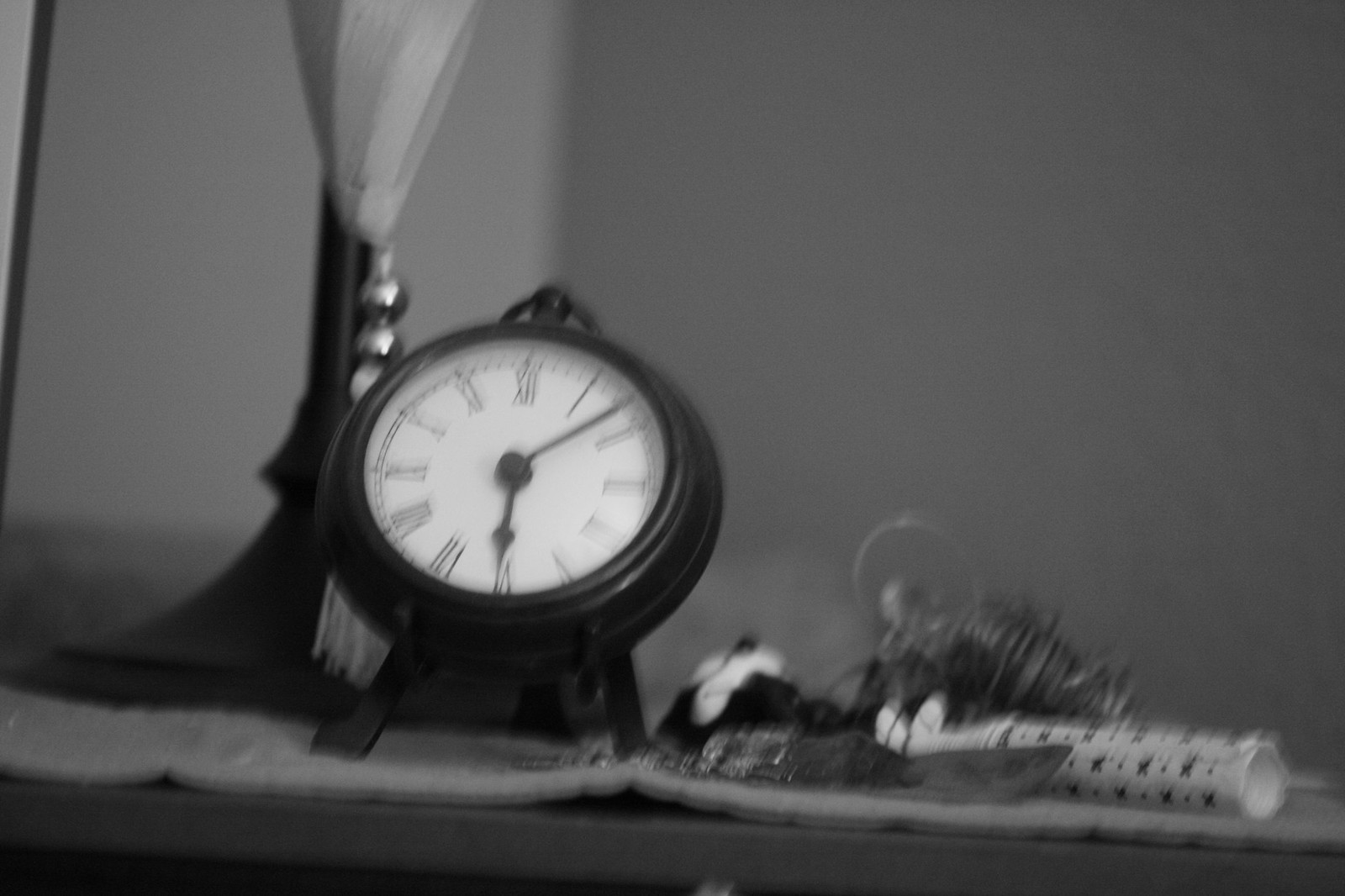This black and white photograph, though slightly out of focus, provides a nostalgic glimpse into a carefully arranged setting atop a dresser, vanity, or desk. Central to the composition is a classic black clock, distinguished by its sturdy black legs and matching black top. The clock's white face prominently displays black Roman numerals, accompanied by black hour and minute hands. In the background, a curtain adorned with beaded fringes adds a touch of elegance and texture to the scene. To the right of the clock, a black stand with a slender pole suggests the presence of a lamp. The backdrop consists of white or gray walls, contributing to the overall muted and timeless atmosphere. Scattered near the clock, a few indistinct items lie partially out of focus, enhancing the authenticity and lived-in feel of the vignette.